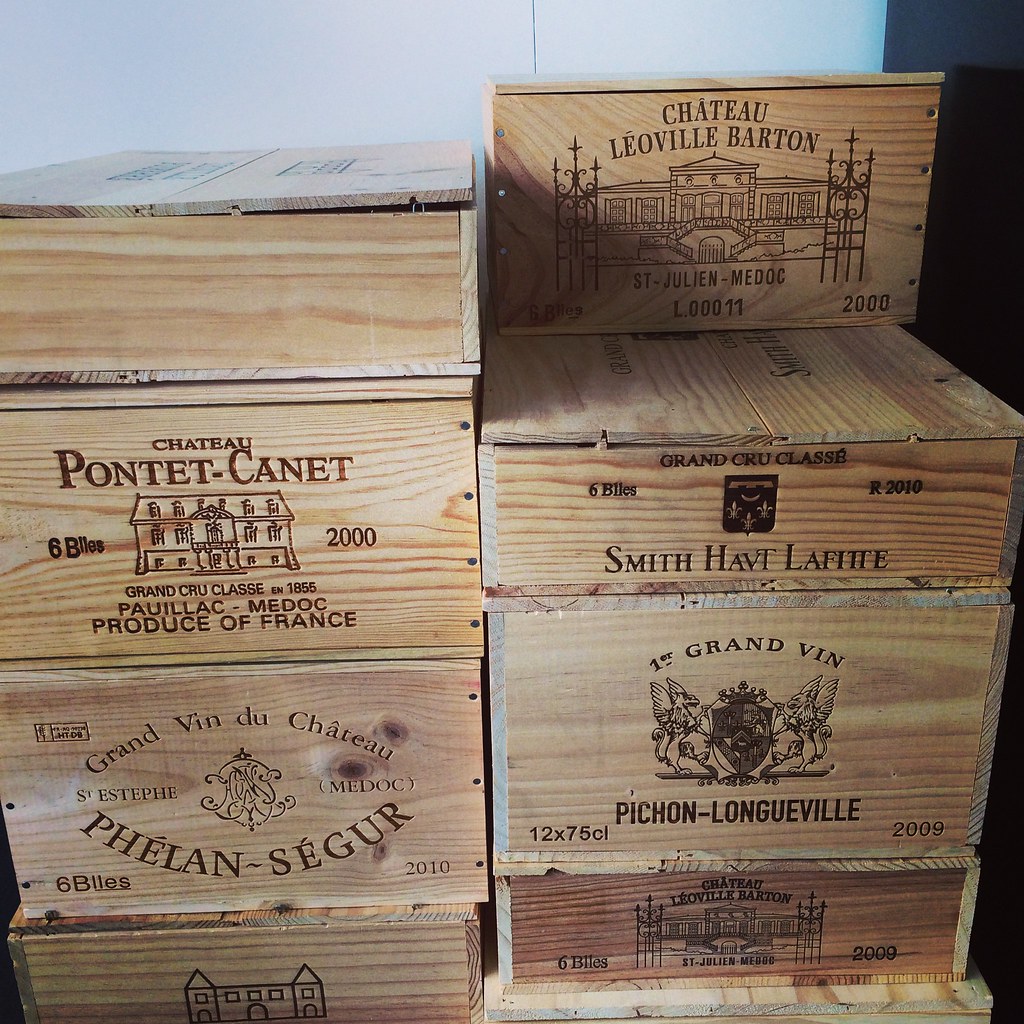This color photograph captures a stack of wooden wine crates, likely French, positioned centrally against a white background wall in what appears to be a warehouse setting. Each crate, made from light-colored wood, is imprinted with various vineyard names, dates, and detailed illustrations or crests. From top to bottom, the visible crates include:

1. Chateau Leoville-Barton, Saint-Julien-Médoc with identifying code L00011 and the vintage year 2008.
2. Smith Haut Lafitte, First Grand Vin Pinche en Longue, marked 2009, featuring a crest with griffins and shield.
3. Chateau Lavaubertin, vintage 2009.
4. Chateau Pont des Canettes, dated 2000, with an illustration of a manor and "Product of France" inscribed.
5. A second crate, noted to be Chateau Lavaubertin, also marked with the year 2000.
6. Grand Vin Château Phelan Segure, dated 2010, with calligraphy-like script at its center.

The crates are closed and neatly stacked, with each displaying distinct branding, including vineyard names, vintages, and various labels and emblems indicative of their prestigious origins. The overall setting emphasizes storage and the organized, cataloged nature of these valuable wine consignments.